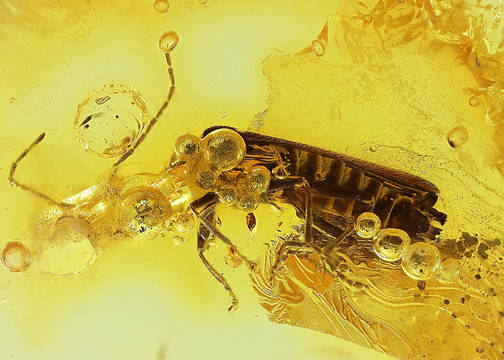This is a color photograph depicting an ancient beetle fossil encased in yellow amber. The amber exhibits varying shades of yellow, transitioning from a lighter hue on the left to a darker tone on the right. The insect, centrally positioned in the image, appears brown with multiple legs and is viewed from the side. Notably, the beetle's segmented rear part is more visible towards the right, while its head is somewhat obscured by bubbles near the upper left portion. The insect has two thin antennae, which are visible towards the upper left of the image. Surrounding the beetle within the amber are numerous bubble-like structures, particularly concentrated around the head and abdomen. These bubbles contain preserved parts of the beetle, adding intricate detail to the fossilized scene.